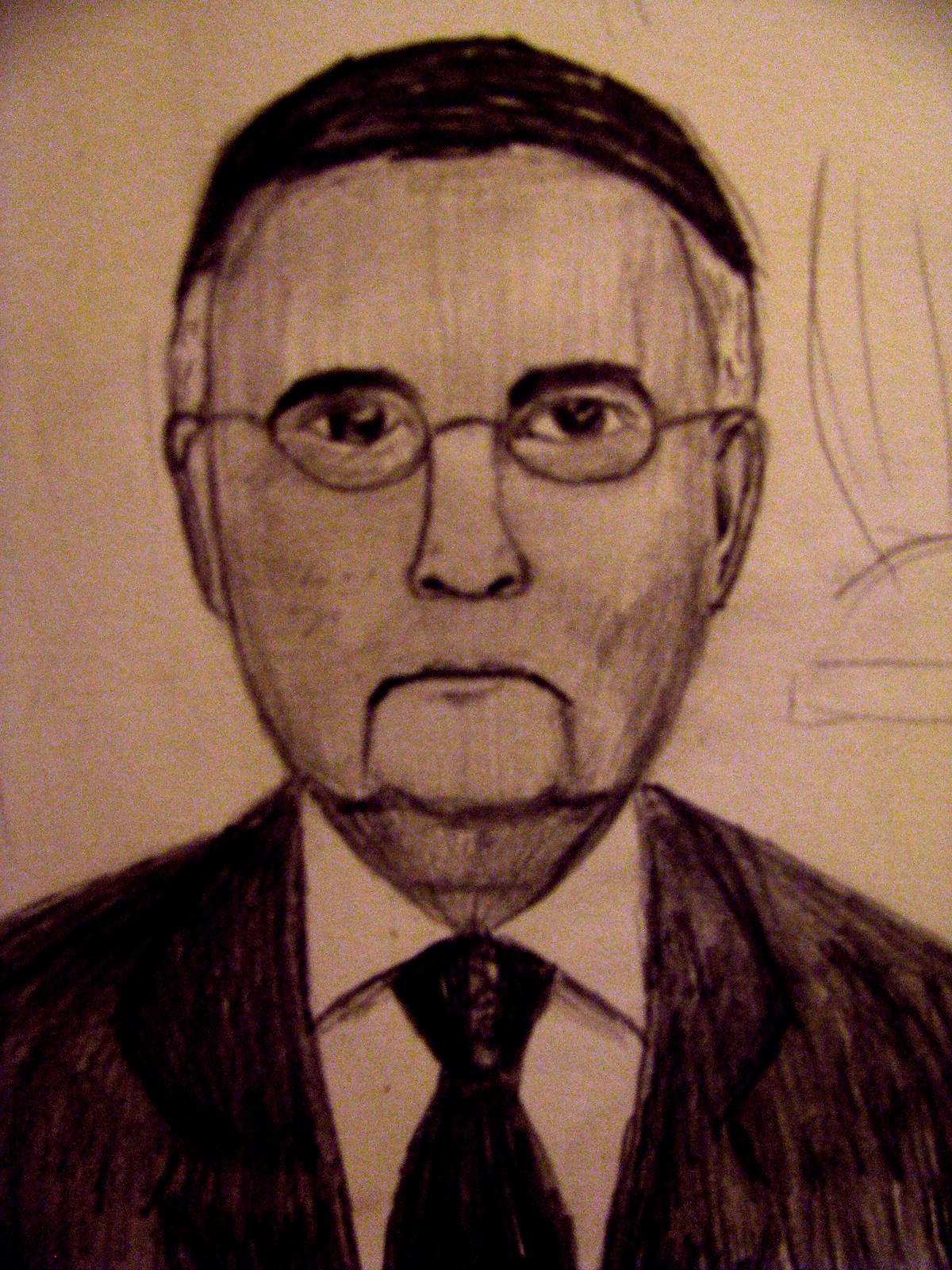This detailed black and white pen illustration depicts a character resembling a puppet. The figure stands against a plain white background, dressed formally in a black suit paired with a white shirt and a black tie. The puppet-like person has distinguishing facial features, including lines marking the contours of the face, giving it a carved appearance. They wear glasses and have short hair on the crown of the head, with white hair framing the sides. Additionally, the character's cheeks are shaded and adorned with freckles, enhancing the puppet-like semblance.